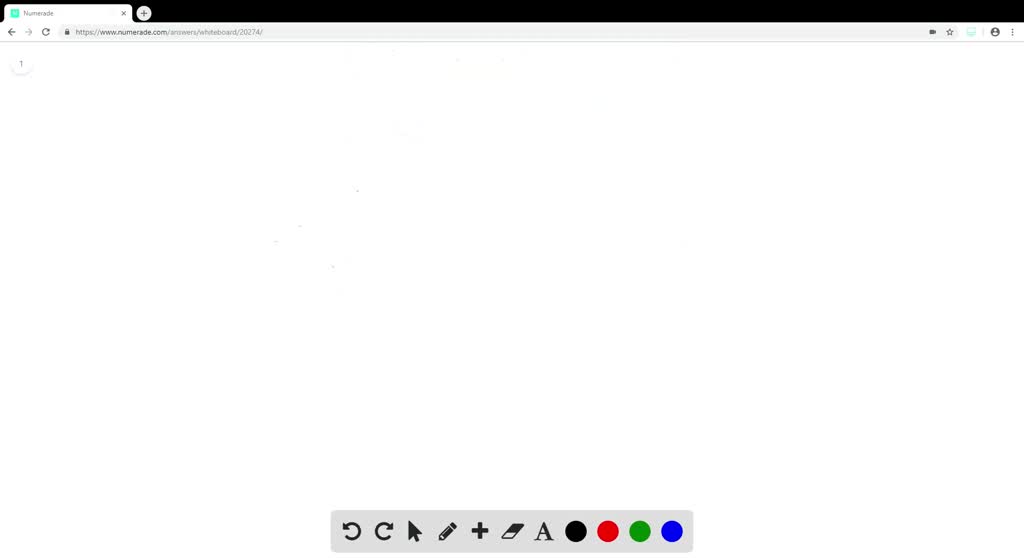The image captures a screenshot from the Google Chrome browser, presenting a website oriented towards digital art creation. The dimensions of the screenshot are notably wider than it is tall, with the exact width challenging to ascertain due to three edges—left, right, and bottom—blending into a white background.

At the very top of the screenshot, the browser's tab bar, set against a black background, is visible. Only a single tab is open, characterized by a white background, an 'X' on the right for closing, and a teal icon on the left. The website name begins with an 'N' in small black text, though it is not entirely legible. Adjacent to the tab, the typical circle icon with a black plus sign is seen, indicating the option to open a new tab.

Below the tab bar, the standard control panel of the browser is displayed, featuring icons for back, forward, and reload functionalities. The address bar showcases the website currently being browsed, with icons for managing favorites on the right, including the familiar star symbol.

The main content area of the browser is blank except for a centered toolbar at the bottom. This toolbar offers various digital art tools, including a pencil, an eraser, a text addition option, and several color selection choices, hinting at the website’s function as a platform for creating or editing art.